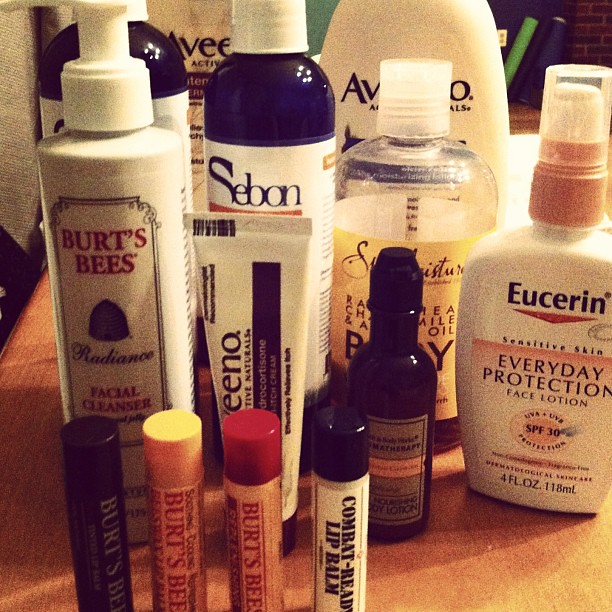The image showcases an assortment of skincare products and lip balms neatly arranged. Starting from the left, the image displays a container labeled "Burt's Bees" followed by the text "Facial Cleanser," indicating it is a facial cleansing product. Next to it is a bottle labeled "Saban," partially obscured by another container labeled "Aveeno." To the right of these, there is a product from "Eucerin," clearly marked "Sensitive Skin" and "Day Protection." Additionally, in the foreground, there are four lip balms aligned side-by-side in a vertical position. Three of these are from "Burt's Bees," while the fourth, at the far end, is labeled "Combat Ready Lip Balm." The image primarily focuses on personal care products, emphasizing facial skincare and lip care items.